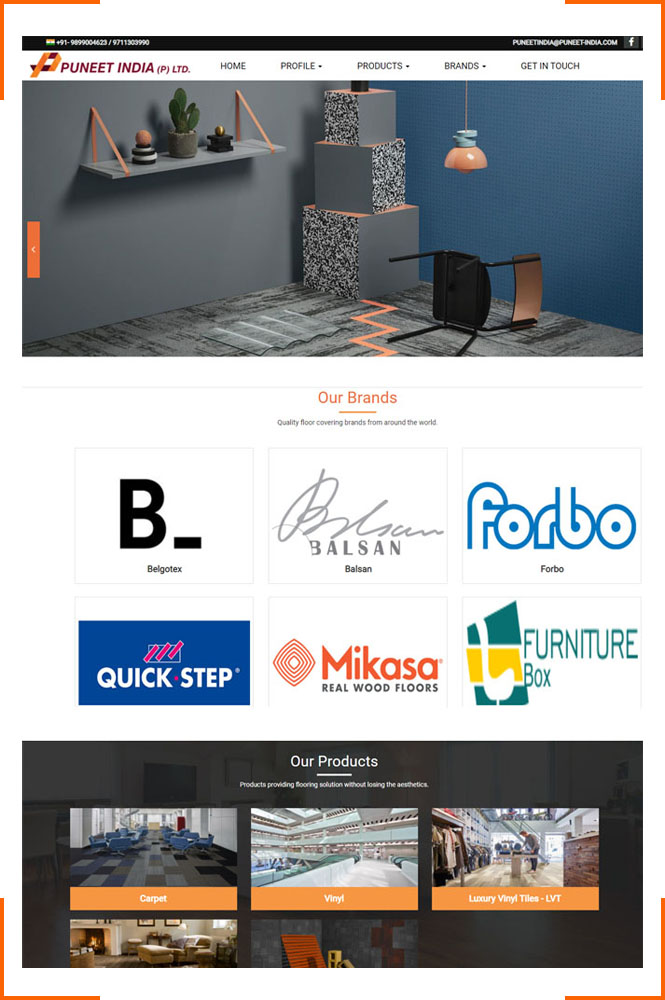The image showcases a website interface, framed by orange brackets in each of the four corners. At the top right of the website, there's an email address: "PunoIndia@PuneIndia.com," accompanied by a small Facebook logo. On the top left, there's a display of numbers resembling a phone number, flanked by a small Indian flag icon on the left. Below this, the website header features the text "Pune India PLTD" alongside a logo designed with an orange and red 'P'.

Just beneath this header, there are navigation tabs categorized as Home, Profile, Products, Brands, and Get in Touch. Central to the webpage is a striking image depicting an overturned chair against a backdrop that transitions from a gray wall to a blue wall. The gray wall hosts a shelf adorned with a pot containing what appears to be a cactus.

Further down, centrally located on the page, are six boxes with the heading "Our Brands" above them. At the bottom of the image, there's a section labeled "Our Products" featuring three boxes, which are classified as Carpet, Vinyl, and Luxury Vinyl.